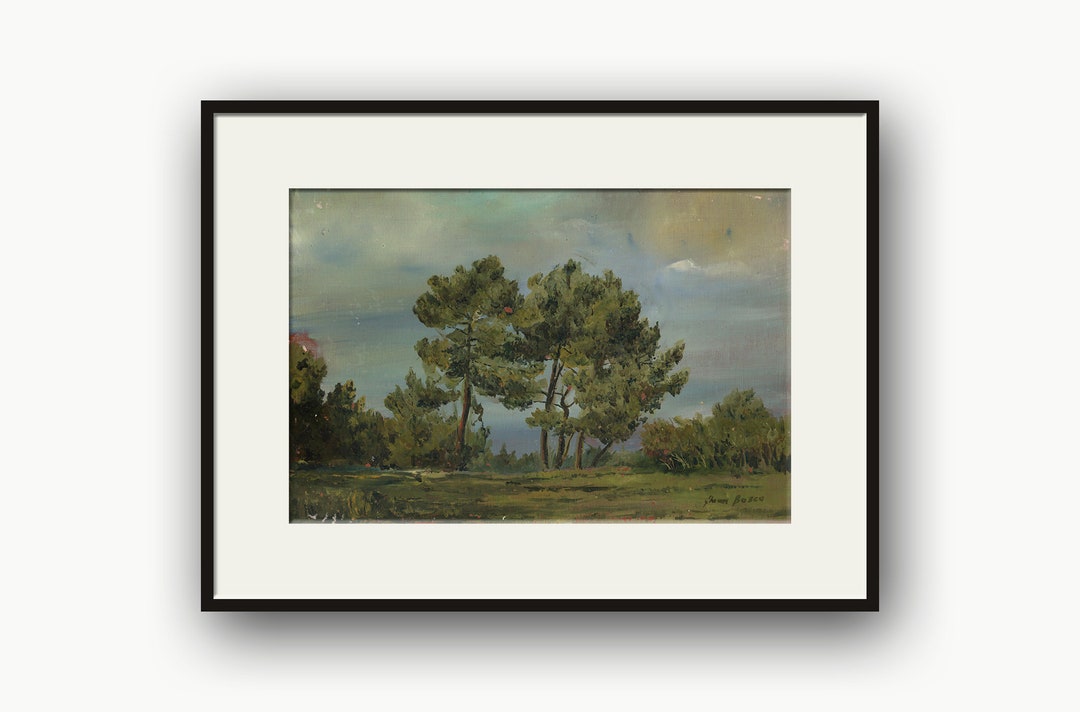The image is a photograph of a painting displayed on a white wall. The painting is encased in a narrow black frame with a white mat, and a slight shadow is cast around it. This pastoral scene depicts a mix of striking elements: lush grass dominates the foreground, transitioning to a more barren look despite its verdant hue. Central to the image is a cluster of five tall deciduous trees, flanked by shorter and thicker vegetation on either side, with some pink hints on the left possibly from a flowering bush. The background features a faint, bluish-gray outline of distant hills or a mountain range, adding depth to the composition. The sky above is predominantly gray and cloudy, accentuating a moody, overcast ambiance, with patches of blue peeking through. The painting bears a signature in the lower right corner, although it's not entirely legible.